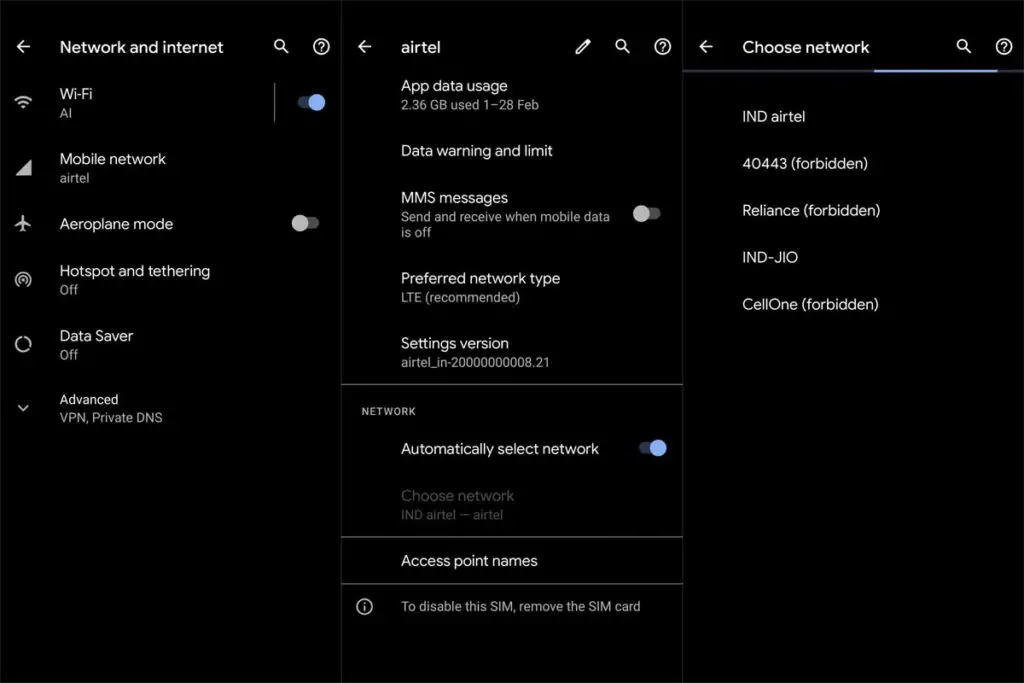**Detailed Screenshot Description: Network and Internet Connection Status**

This screenshot provides a detailed overview of the network and internet connection settings on a mobile device.

**First Section: Wi-Fi and Mobile Network Status**
- **Wi-Fi Status:** The Wi-Fi is currently enabled and connected to a network named "AI."
- **Mobile Network:** The mobile network service provider is Airtel.
- **Aeroplane Mode:** Aeroplane mode is turned off.
- **Hotspot and Tethering:** Both features are turned off.
- **Data Saver:** Data Saver mode is turned off.
- **Advanced Options:** There are drop-down menus available for VPN and private DNS settings.

**Second Section: Airtel Data Usage and Settings**
- **Header:** Displays "Airtel" with an icon of a pencil for editing, a search bar, and a help icon (a question mark inside a circle).
- **Data Usage:** The app data usage for the period is 2.36 GB, calculated from February 1st to February 28th.
- **Data Warning and Limits:** There is an option to set a data warning limit.
- **MMS Messages:** Sending and receiving MMS messages when mobile data is off is disabled.
- **Preferred Network Type:** The device is set to use LTE, which is the recommended network type.
- **Settings Version:** Listed as Airtel_in-20000000008.21.
- **Network Selection:** Automatically select network is toggled on.
- **Access Point Names (APNs):** Accessible but not detailed in this screenshot.
- **SIM Management:** To disable the SIM, it instructs to remove the SIM card.

**Third Section: Available Networks**
- **IND Airtel:** Identified with the code 40443, marked as forbidden.
- **Reliance:** Marked as forbidden.
- **IND-JIO (Cell 1):** Also marked as forbidden.

The layout includes a thin white line separating different pieces of information, ensuring clarity and visual separation of settings.

This detailed caption accurately reflects the intricate settings and options visible in the screenshot, providing comprehensive insights into the device's network and internet configuration.